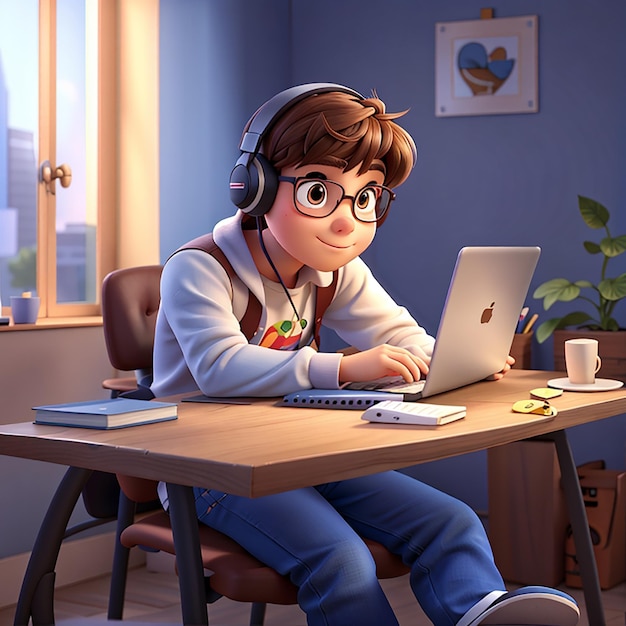In this detailed 3D cartoon-style graphic reminiscent of Disney animation, a young boy or teenager is depicted sitting at a wooden desk. His short brown hair with bangs partially covers his forehead, and he is wearing glasses and headphones that sit over his ears. He dons a white long-sleeve shirt with a logo, a white and maroon hoodie, blue jeans, and blue sneakers.

The desk, made of wood, holds an Apple laptop with the recognizable logo. Nearby, there's a blue notebook, a white coffee cup on a plate, a potted plant, and a pencil holder with pencils. A book and some indeterminate yellow items are also scattered on the desk. The boy sits on a brown chair in a room with light blue walls, where a framed portrait hangs; the portrait features a blue and brown image. 

Behind him, a window reveals a cityscape with buildings and a bright blue sky. The desktop scene is bathed in green color tones, contrasting with the calm blue of the walls and outside world.